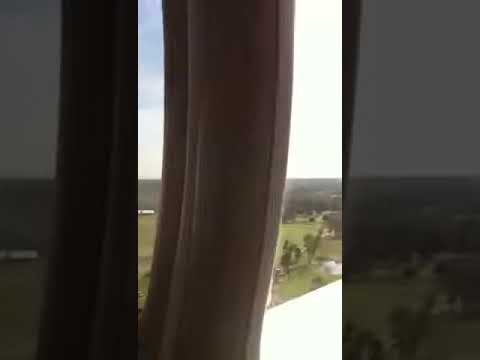The image captures a view through a window adorned with a tan curtain or shade, which is gathered and hangs vertically in the center, dividing the scene into thirds. On both sides of this central curtain, there are darker vertical areas, possibly indicating parts of the window frame or additional drapery. Directly below the curtain, the viewers can glimpse the structure of the building, featuring a white ledge that ascends diagonally. Beyond the window, a picturesque countryside unfolds, showcasing a mix of green fields, sporadic trees, and a distant tree line under a partially cloudy blue sky. The overall scene is accentuated by the contrast between the bright outdoor landscape and the darker indoor elements framing it.